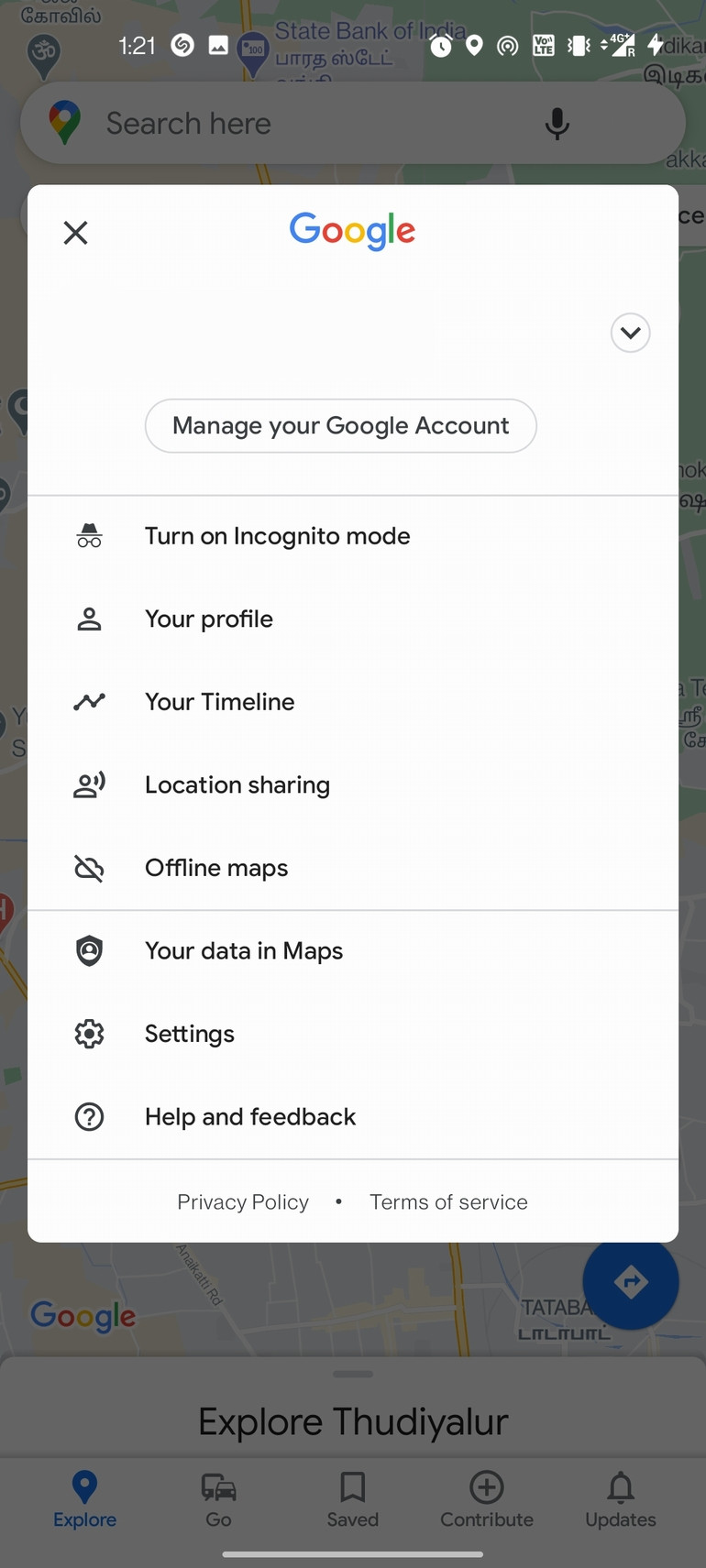The image displays the interface of a smartphone with an active Google search on the screen. The phone's screen is partially blacked out, with a highlighted pop-out area featuring a Google search interface. This pop-out section has a white background prominently showcasing the multicolored Google logo at the top, alongside an 'X' icon on the left, indicating the option to close the screen.

Below the Google logo, centered on the screen, is the prompt "Manage your Google Account." The options under this prompt are listed from top to bottom as follows:

1. "Turn on Incognito mode" - accompanied by an incognito icon to its left.
2. "Your profile" - with a person icon on the left.
3. "Your timeline" - represented by a timeline icon next to it.
4. "Location sharing"
5. "Offline maps"
6. "Your data in Maps"
7. "Settings"
8. "Help & Feedback"

At the bottom of this list, in smaller and fainter letters, are "Privacy Policy" and "Terms of Service."

In the background, faintly visible behind the pop-out screen, appears to be a map interface, suggesting that this screen is possibly a menu popped out from the Google Maps application.